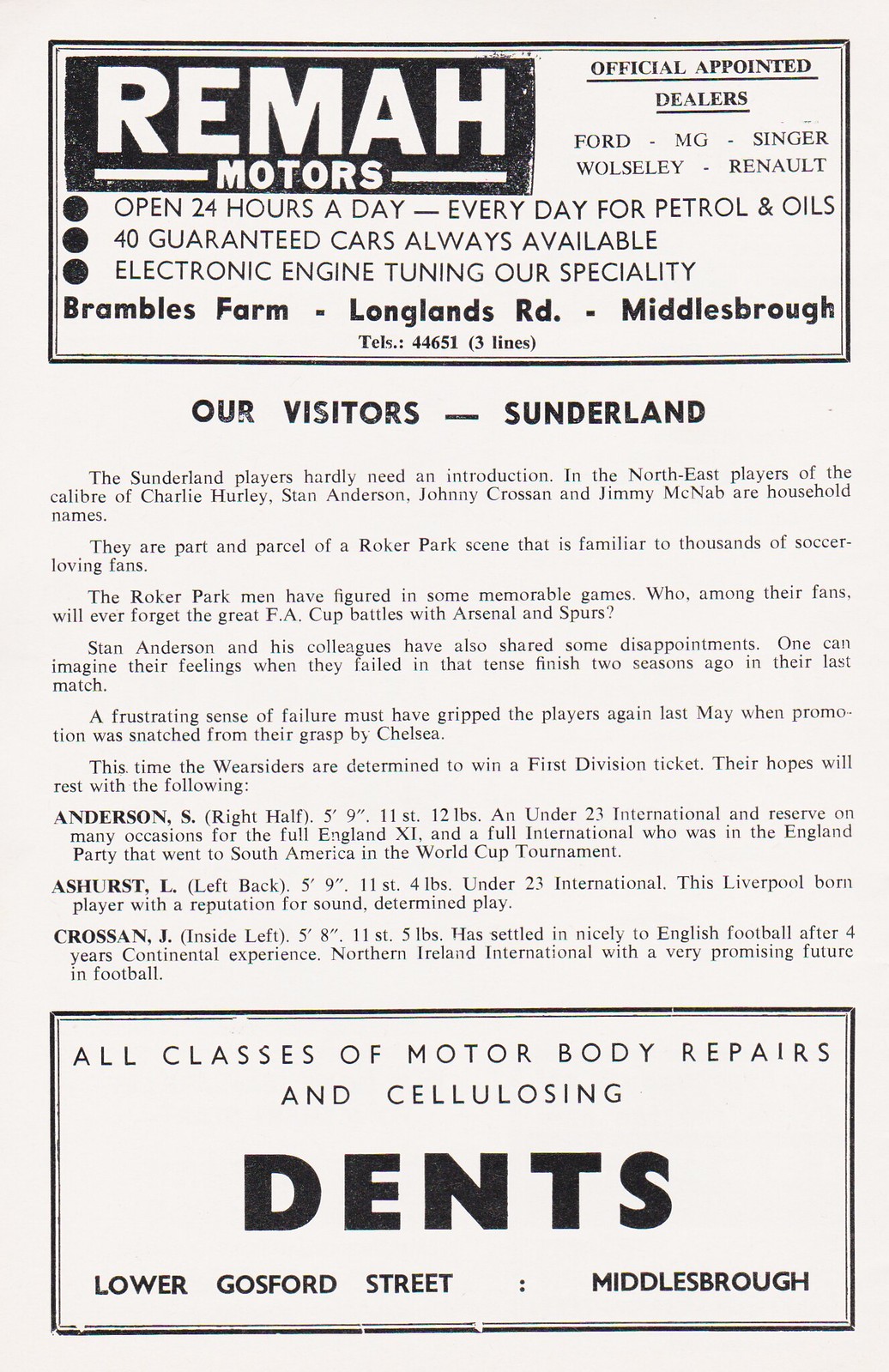This detailed page from a soccer program guide features advertisements and information seamlessly integrated within the overall layout. At the top, there's a rectangular black-and-white advertisement for Rima Motors, which provides insights into their offerings: open 24 hours daily, they specialize in petrol, oils, and electronic engine tuning. Located at Bramble Farm, Longwoods Road, Middlesbrough, Rima Motors is an official dealer for prominent car brands such as Ford, MG, Singer, Wolseley, and Renault, boasting 40 guaranteed cars always available.

In the central section, the headline "Our Visitors: Sunderland" introduces the visiting team with a detailed narrative. The text briefly celebrates the well-known Sunderland players, highlighting their strong reputations in the Northeast. Renowned footballers like Charlie Hurley, Stan Anderson, Johnny Carson, and Jimmy McNabb are described as household names. The text continues with listings and specific details of three Sunderland players: S. Anderson, positioned as right half at 5'9" weighing 12 pounds; L. Ashhurst, a left-back also at 5'9"; and J. Crossing, the inside left at 5'8".

Concluding the page is another rectangular black-and-white advertisement for Dents, a business offering comprehensive motor body repairs and cellulosing services. Located on Lower Gosford Street, Middlesboro, Dents is likely a separate entity from Rima Motors, providing specialized repair services for various motor classes.